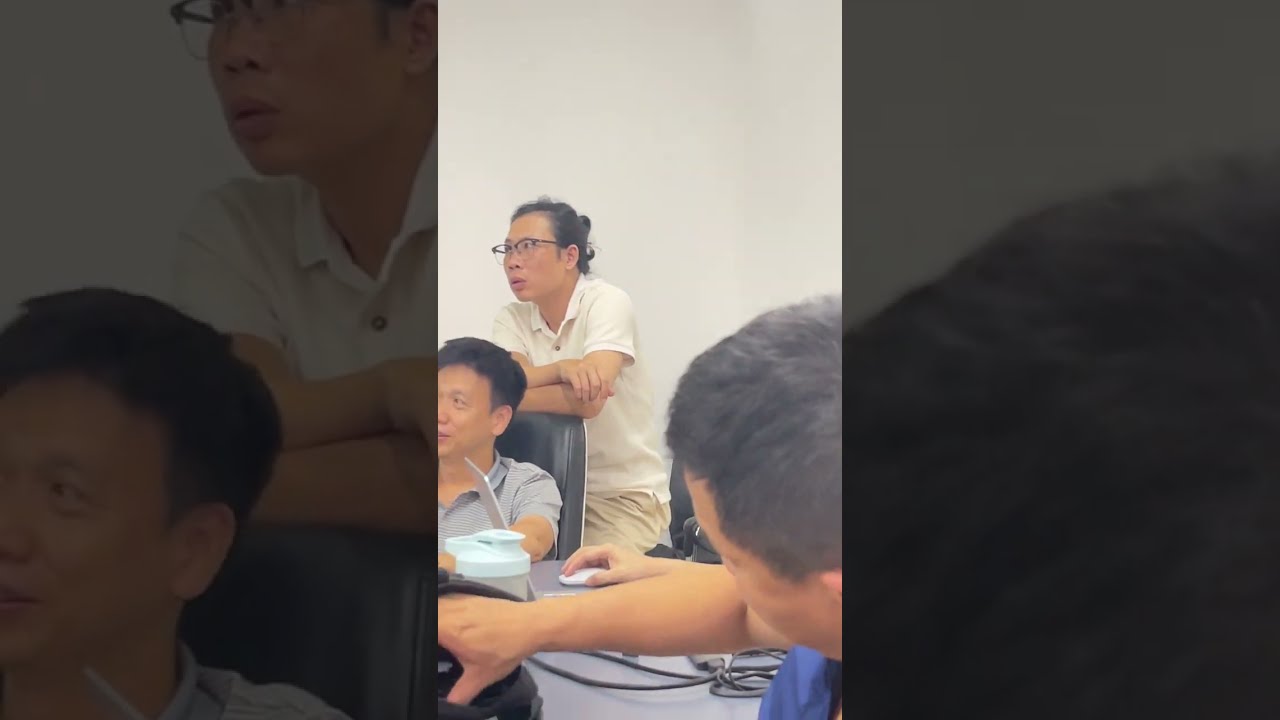The image showcases a detailed, indoor setting featuring three Asian individuals around a conference table. Centered in portrait orientation, it appears to be a cell phone photograph displayed within a landscape inset of the same photo.

On the right side in the foreground, a man wearing a blue shirt with short black hair leans forward. He extends his arm towards the table, reaching for an object, possibly headphones, connected by a black cord. Only the top of his head and his hand are clearly visible in the image.

To the left, a man in a gray or blue striped polo shirt occupies a black chair. Part of his face is visible, displaying a slight smile. He looks upwards towards an unseen object or person off-screen, as does the man standing behind him.

Behind this seated man, a middle-aged woman in a white polo shirt with tan pants and wearing dark-framed glasses stands with her arms resting on the back of his chair. Her hair is pulled back in a ponytail, and she too is focused on the same point beyond the frame.

The background is a flat, beige wall, while the conference table, covered in a grayish-blue surface, holds various cords, possibly laptops, and a water bottle. An almost invisible extra hand, hinting at another person, can be seen slightly behind the man in the blue shirt, adding to the image's depth and dynamic.